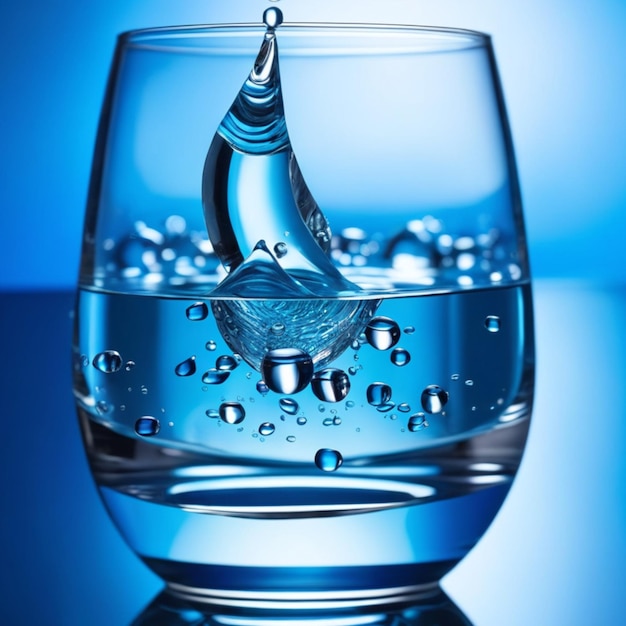The image is a detailed, close-up photograph of a transparent glass, half-filled with water, capturing a dramatic splash as a droplet falls into it. The background is a lighter blue, and this blue hue reflects through the clear water, tinting the scene in various shades of blue. The glass, which has a cylindrical shape with a curved base resembling a stemless goblet, stands on a blue surface, reinforcing the cool color scheme. As the droplet connects with the water, bubbles form and scatter, with several large ones mimicking the glass's shape and slightly floating at the top. The composition focuses centrally on the glass, revealing intricate details like the suspended droplet frozen in mid-air, bubbles within the water, and the dynamic interplay between motion and stillness, all tinged in blue gradients.